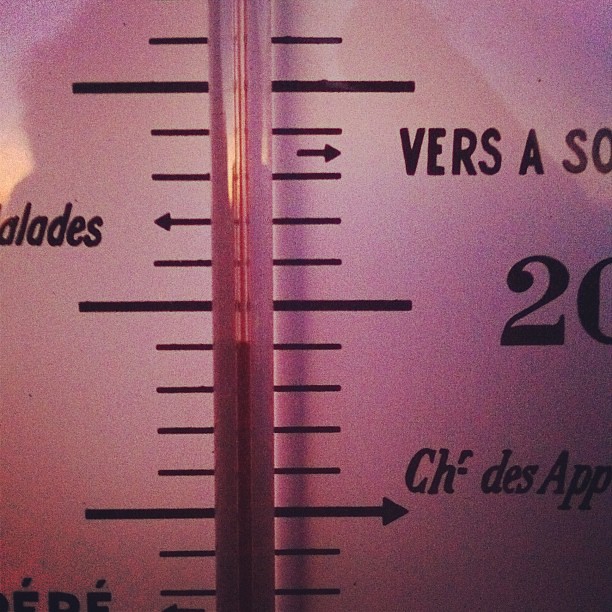A tightly-cropped image of what appears to be a thermometer, displaying a temperature just below 20 degrees Celsius, estimated at around 18 degrees. The surface of the thermometer is marked with increments every 10 degrees, with longer, darker lines at intervals of 10 and 30. French words are visible on both sides of the instrument, including 'vers,' although the rest of the text is obscured. The image is dimly lit, likely due to the shadow of the photographer obstructing the light source.